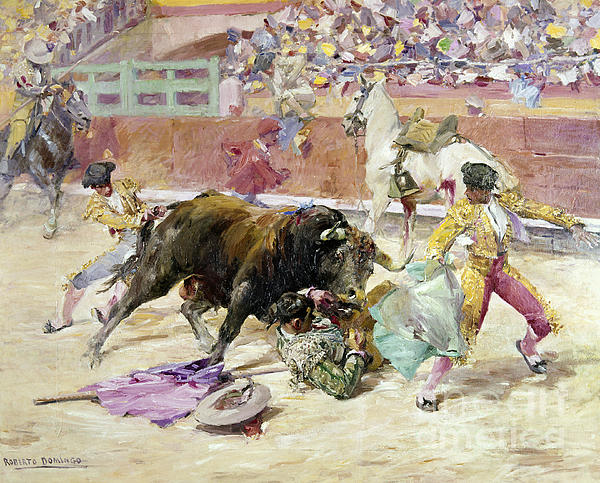This captivating watercolor painting signed by Roberto Domingo in the bottom left corner, vividly portrays the intensity of a bullfight in a surreal, dreamlike style. Dominating the scene is an oversized, powerful brown bull with blood-streaked horns, indicating its upper hand in the fray. A fallen bullfighter lies defenseless on the ground, his hat cast aside, possibly impaled by the bull. 

Two other bullfighters in ornamental traditional attire, resplendent in pink and gold, desperately work to control the ferocious animal—one pulls its tail while the other attempts to distract it from the front. The background is populated with details such as a white horse, seemingly injured, and a black horse ridden by another participant in red clothing. These figures suggest the chaotic and collaborative efforts involved in the bullfight.

The audience, though not individually distinguishable, forms a curious and ethereal crowd, their vague forms rendered with dreamlike abstraction. The painting employs a striking palette of colors including black, white, brown, pink, red, yellow, gold, green, blue, and purple, adding to its rich, almost mystical character. Despite the palpable tension and violence, the artwork maintains a sense of fluid, almost fantastical movement, underscoring its professional and imaginative craftsmanship.